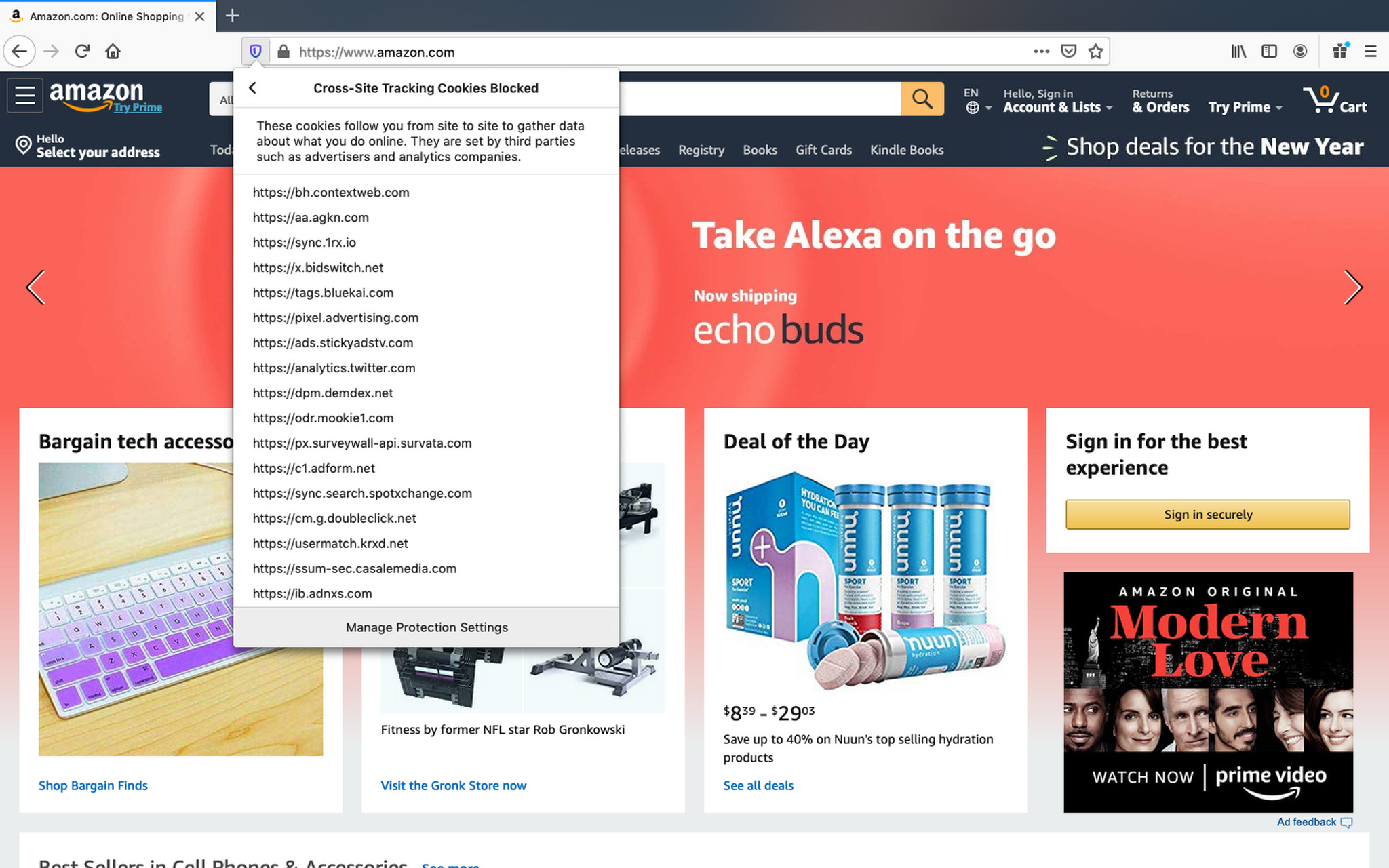This is a detailed screenshot of the Amazon.com landing page. Prominently featured is the browser's URL bar on the left, where a badge icon is highlighted. This badge opens a drop-down menu detailing the blocking of cross-site tracking cookies. These cookies, which are set by third parties such as advertisers and analytics companies, monitor user behavior across different websites. The drop-down menu lists approximately 20 different tracking cookies, illustrating the extent of online tracking.

Below the URL bar is Amazon's full menu bar, offering various options including 'Registry', 'Books', 'Gift Cards', and 'Hello, select your address'. This comprehensive menu also includes account information options.

Further down, an orange banner invites users to "Take Alexa on the go," featuring a promotion for Echo Buds. Below this banner are four tiles: the first tile promotes bargain tech accessories, the second is for the Gronk Store which appears to sell gym equipment, the third highlights Noom Fitness Salts as the "Deal of the Day," and the fourth, located at the bottom right, encourages users to sign up for the best experience. Additionally, there's a promotion for "Amazon Original Modern Love" with an option to "Watch Now on Prime Video."

This detailed view offers insights into both the tracking mechanisms operating on the site and the various shopping and service options available on Amazon's landing page.